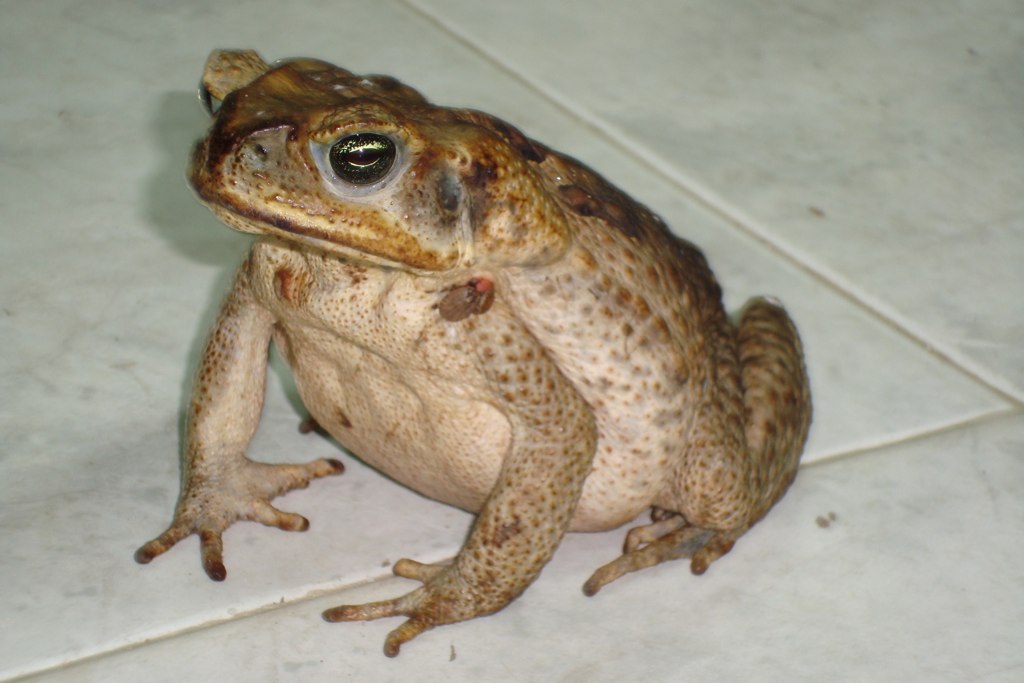The image depicts a large toad seated upright on its back legs, with its front legs and long fingers splayed out on an off-white, marble-like bathroom tile floor. The background and underneath the toad feature hard tile flooring with visible creases where the tiles fit together, extending from the bottom left corner across to the right edge, and then up towards the top edge of the image, which is a horizontal rectangle. The toad's belly is a whitish or very light cream color, contrasting with its orangish-brown, burnt-looking back, adorned with warts. The toad's eyes are circular and bulbous, with a golden hue. Its legs are long with webbed feet at the back, and its front legs also exhibit long fingers. The toad is facing to the left and slightly towards the camera, showcasing its black eyes and darker-toned nose. This photograph captures the toad in the middle of the picture, creating a detailed and vivid portrayal of the amphibian in its environment.